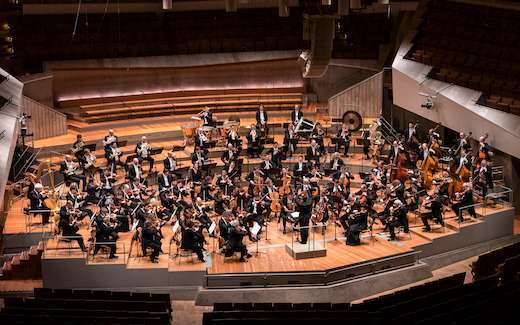This horizontal, rectangular image showcases a meticulously staged orchestra poised for what seems like a rehearsal in a grand concert hall or a large arena with a circular setup. The orchestra, composed of numerous musicians mostly seated, occupies a prominent, slightly raised stage adorned with orange tones and bordered by elegant pink marble settings. At the forefront stands a conductor on a small podium, directing the ensemble, with the percussion section stationed at the back and possibly some standing musicians playing specific instruments.

The concert hall emanates a sense of grandeur with empty, well-constructed seats encircling the stage—these seats, rising in tiers like bleachers, all feature backrests and remain unoccupied, suggesting either a rehearsal or preparation before the main event. The photograph, snapped from a high vantage point at the back of the stage, captures the pristine hardwood flooring, the impressive lighting, and the intricate detail of the arena’s architecture, including steps leading up to an empty second stage behind the orchestra.